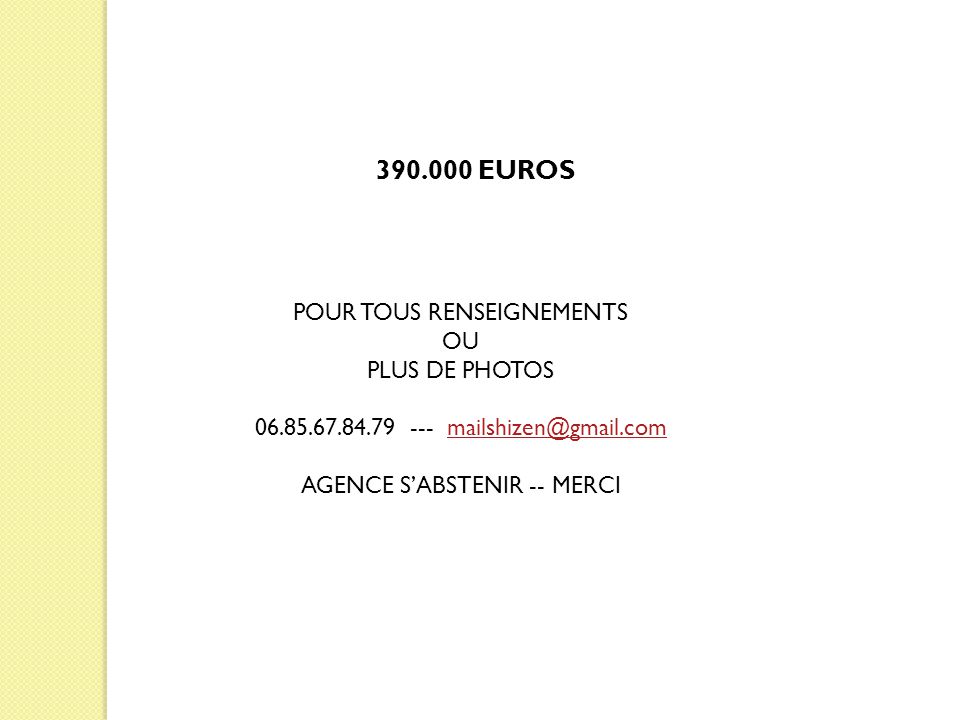This image features a simple, uncluttered design with a white background. A thin yellow vertical strip runs along the entire left edge, taking up roughly 10% of the image width. At the top center of the image, bold black text displays the amount "390.000 euros" (using a dot as the thousands separator, typical in European formatting). Below this, French text reads "Pour 2 raisons malts ou plus de photos," which roughly translates to requesting additional pictures for validation. Following this, in black text, is a phone number punctuated with dots: "06.85.67.84.79". Next to the phone number are three dashes, succeeded by a red hyperlinked email address "mailchizin@gmail.com". At the bottom of the image, in black uppercase letters, it reads "AGENTS S'ABSTENIR," followed by "MERCI" signifying a polite closure. The entire text is presented in a clean and professional manner.